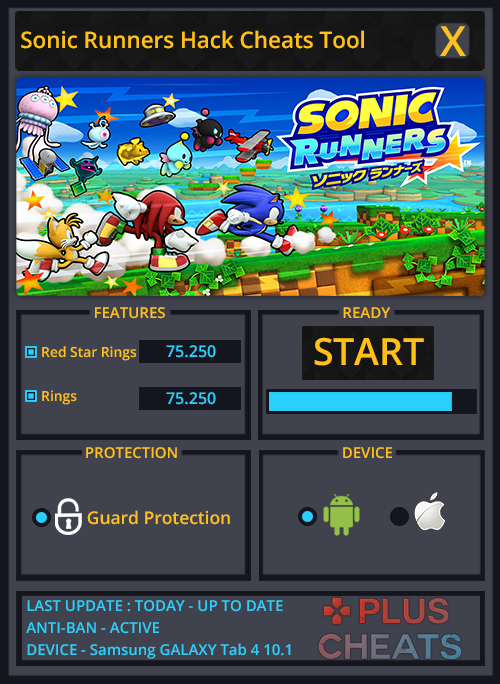Screenshot of a Computer Game Interface for "Sonic Runners Hack Cheat Tool":

The image showcases a computer video game interface titled "Sonic Runners Hack Cheat Tool," indicated prominently in a yellow bar at the top, accompanied by a yellow 'X' on the right side for closing the window. Below this title, a rectangular banner features the "Sonic Runners" logo in blue and yellow, accompanied by text in Asian script beneath it.

The central part of the banner displays Sonic the Hedgehog characters sprinting from left to right. Sonic leads the group in the middle, trailed by a red character and a yellow character. Additional characters can be seen flying overhead, set against a backdrop of a vibrant blue sky, water bodies, and lush greenery, suggesting they are running across a bridge.

The lower section of the interface features a gray background with various functional boxes. On the left side, there's a box labeled "Features" at the top, listing "Red Star Rings: 75.250" and "Rings: 75.250." To the right, a box marked "Ready" and then "Start" is positioned above a blue energy bar. 

In the bottom left corner, a box titled "Protection" showcases a padlock icon and the text "Guard Protection" in yellow. The bottom right corner contains a "Device" label in yellow, displaying a green alien icon with a blue circle next to it and a white Apple symbol with a black circle.

At the very bottom of the interface, a lengthy rectangular box provides additional information, stating "Last Update Today," "Up to Date," "Anti-Ban Active," and "Device: Samsung Galaxy Tab." The box is capped off with “Plus Cheats” in a red and blue color scheme in the bottom right corner.